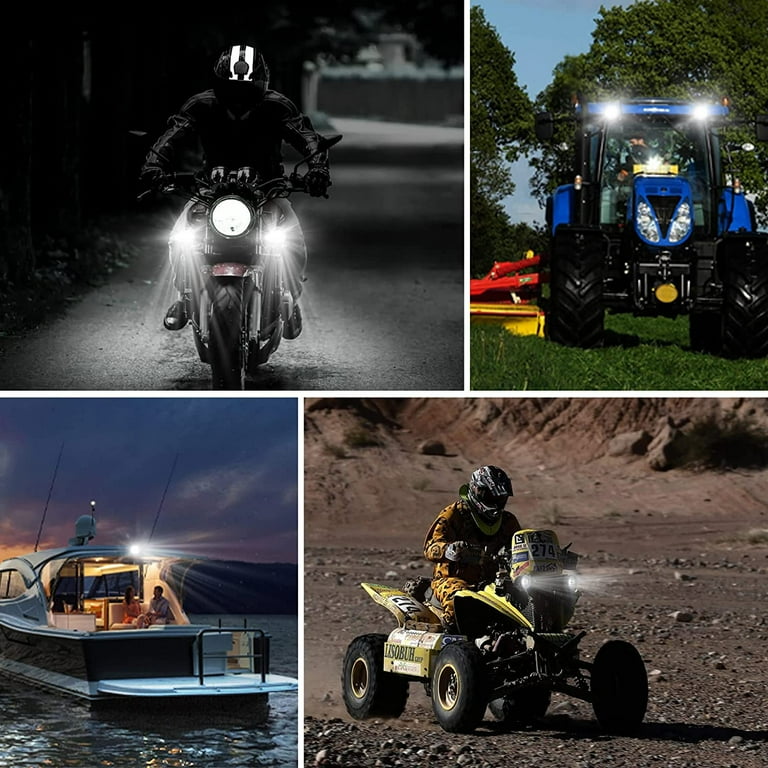The image is a detailed mosaic divided into four equally sized sections, each portraying a different type of vehicle in various outdoor settings. 

In the top left corner, there is a motorcycle facing the camera with its lights on, situated on a darkened road. The rider is dressed in a black jacket, blue jeans, and black shoes, with a distinctive black helmet adorned with two thick white stripes and a thinner black stripe down the center.

The top right corner features a blue tractor with large wheels, positioned in a grassy field. The tractor's headlights are also illuminated, casting light on an adjacent implement near the front right tire, which is yellow at the base and red on top, potentially an oversized lawnmower or tiller. Green trees form the backdrop.

In the bottom left corner, a sleek yacht is anchored on a serene lake during sunset, with pink and purple hues in the sky. The yacht, black on the body with a white deck and top, has a single headlight turned on. A man and a woman sit on a couch at the back of the yacht, enjoying the picturesque scene with mountains in the background.

The final section, in the bottom right corner, shows a man riding a yellow four-wheeler in a gravel quarry, competing in what appears to be an ATV event. His vehicle sports the number 272. He wears a dark helmet with a black visor and a jumpsuit featuring a leopard print pattern. The atmosphere is dusty and brown, consistent with the quarry surroundings.

Overall, the mosaic showcases various recreational vehicles captured in vibrant outdoor settings, ranging from grassy fields and lakes to dark roads and gravel quarries.